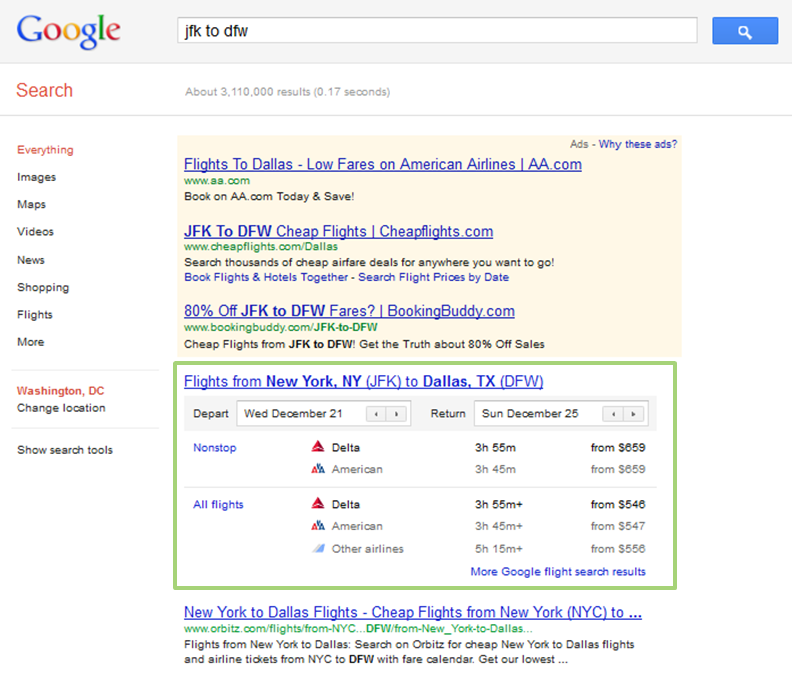A detailed screenshot of a Google search results page for flights from JFK to DFW (New York to Dallas). At the top, the familiar Google logo in its vibrant, multicolored letters is prominently displayed above the search bar, which contains the query "JFK to DFW." The search yielded approximately 3,110,000 results in 0.17 seconds.

The first visible result is an advertisement, highlighted in yellow. Advertising low fares on American Airlines with tags like "cheap flights" and "cheapflights.com," two prominent offers catch the eye: one from Booking Buddy promoting 80% off JFK to DFW fares.

Beneath the ads is a highlighted white box with a distinct green border, detailing specific flights from "New York, New York (JFK)" to "Dallas, Texas (DFW) – Dallas-Fort Worth." It outlines departure on Wednesday, December 21st, and return on Sunday, December 25th. The box provides two nonstop flight options from Delta and American Airlines, both with similar durations (Delta: 3 hours 55 minutes, American: 3 hours 45 minutes) and starting prices from $659.

Further down are all available flights, including those with one stop or more from Delta, American, and other airlines. Similar in-flight durations for Delta and American are stated (Delta: 3 hours 55 minutes, American: 3 hours 45 minutes), but the other airlines' flights vary significantly, with some taking upwards of 5 hours and 15 minutes.

Pricing for these flights shows Delta at $546, American at $547, and the other airlines slightly higher at $556, emphasizing the inconvenience and higher cost of longer flights with layovers. 

The final result highlighted at the bottom offers cheap flights on ORBITZ.com, advertising potential deals from New York to Dallas.

This comprehensive page layout provides users with a range of options, from nonstop flights with major airlines to more time-consuming and costly alternatives involving multiple stops.